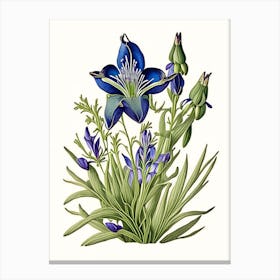This image depicts an intricately detailed painting of a blooming flower arrangement set against a white wall. The central focus is a majestic blue flower with five petals, featuring light purple segments protruding from its center. The flower, emerging from a cluster of vibrant green, sword-shaped leaves, stands out prominently. Surrounding it are multiple smaller, fully-bloomed blue flowers and two buds that have yet to open, adding a sense of anticipation to the scene. The petals and central purple pods create a dynamic visual contrast, while the dense green grass at the bottom frames the composition, extending out from the sides and filling the entire rectangular artwork.